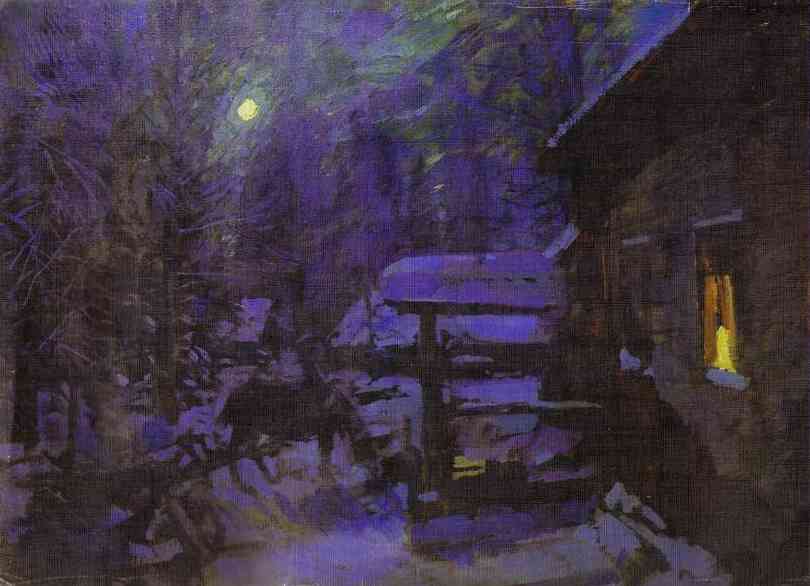This detailed oil painting depicts a serene nighttime winter scene centered around a rustic log cabin-style house situated in a snow-covered forest. The cabin, constructed of brown logs, occupies the right half of the painting. Emanating a warm golden-yellow glow, light spills out from a solitary window on the side of the house. In front of the house, a small woodpile is visible, further emphasizing the rustic winter atmosphere. The cabin features a tiny porch area with snow delicately blanketing its awning.

To the left side of the painting, an animal, possibly a deer or a small horse or donkey, stands amidst the snow, contributing to the tranquil woodland setting. Surrounding the animal, snow-covered trees enhance the wintry backdrop. Tall pine or palm trees frame the background against a clear night sky, where a distinct, round yellow moon casts a gentle glow, creating a subtle interplay of shadows on the snow. The overall color palette of the artwork includes shades of green, brown, purple, blue, black, white, gray, yellow, and orange, which blend harmoniously to convey the peaceful, cold, and quiet essence of the winter night.